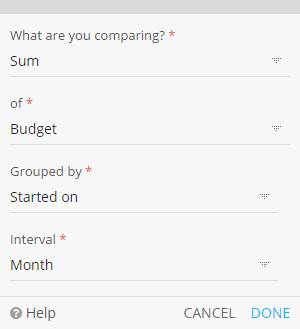Screenshot of a settings menu with detailed options:

The screenshot showcases a settings menu displayed against a light grey background, with a medium grey stripe forming a small band at the top of the frame. The menu features four drop-down options, each accompanied by labels and red asterisks indicating required fields.

1. The first drop-down menu is labeled "What are you comparing?" in thin grey text with a red asterisk next to it. The menu itself is embedded in a light grey line with a downward-pointing arrow made of dots and currently shows the word "SUM."

2. Below this, a similar layout presents the label "OF" in light grey text with a red asterisk, and the drop-down menu displays "BUDGET" in capital letters.

3. Next, the label "GROUPED BY," also marked with a red asterisk, is shown above a slightly truncated drop-down menu that contains the words "STARTED ON."

4. The final option is labeled "INTERVAL" with another red asterisk, and the corresponding drop-down menu reads "MONTH."

A thin grey line separates these options from the bottom section, which includes three elements: "HELP" on the left side next to a grey circle with a white question mark, and "CANCEL" in grey and "DONE" in blue on the right.

This succinct view captures the essential components and layout of the settings menu.